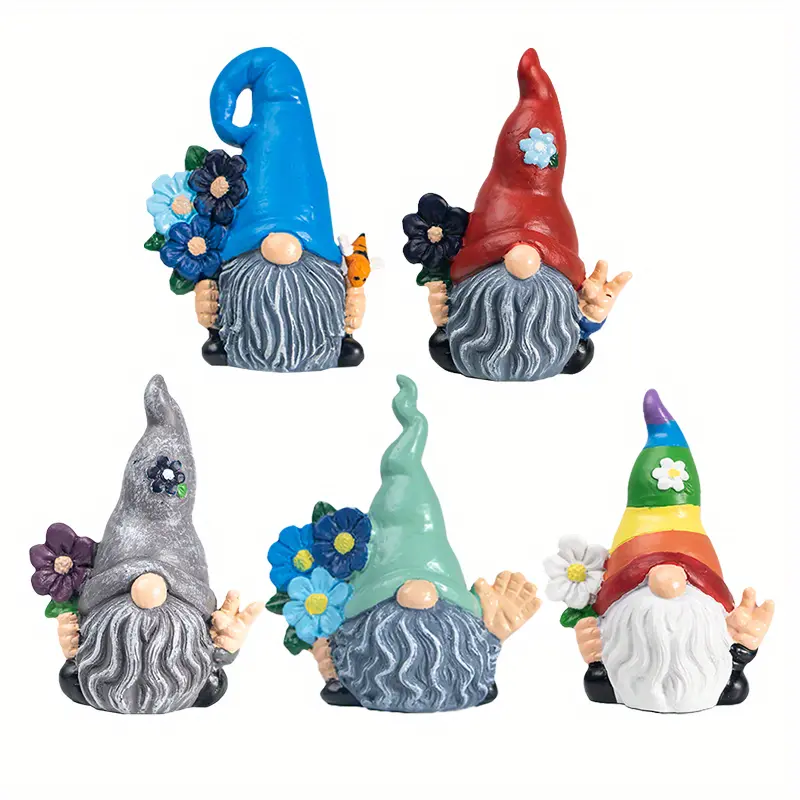This image showcases a charming set of five ceramic garden gnome figurines, each adorned with distinct pointy hats that hide their eyes, leaving only their prominent noses and beards visible. Positioned against a plain white background, the gnomes are arranged in two rows; two on the top and three on the bottom. The top left gnome sports a dark blue hat and a gray beard while holding a dark blue flower. Beside him, the top right gnome has a red hat, a gray beard, and clutches a black flower. On the bottom row, the leftmost gnome features a gray hat and a gray beard, holding a purple flower. The middle gnome on the bottom row possesses a mint green hat, a gray beard, and presents a light blue flower. The rightmost gnome stands out with a rainbow-colored hat embellished with a white flower, accompanied by a white beard and another white flower in hand. Each gnome's other hand is either waving or gesturing, adding a playful touch to their unified yet individually unique designs.